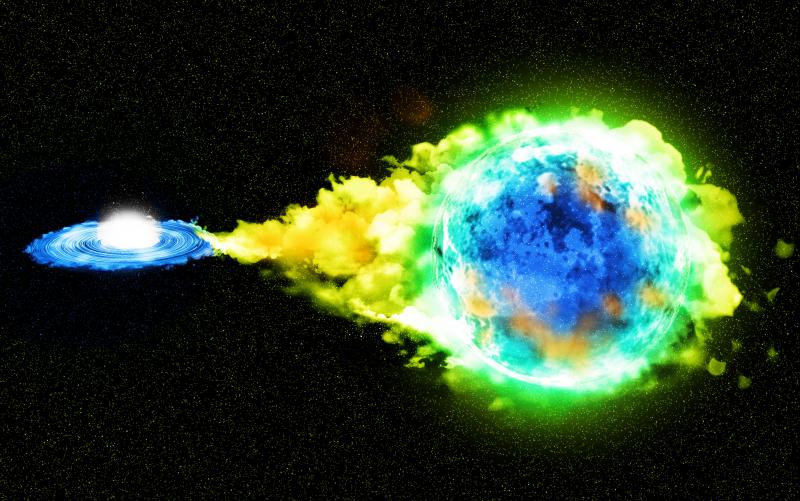The image is a detailed and vivid illustration depicting two celestial bodies floating in space against a backdrop studded with stars. On the right side of the image is a large blue planet adorned with various shades of blue regions. This planet is encircled initially by a green cloud that transitions to a yellowish hue towards its outer edges. This cloud appears to flow and connect towards a second celestial object on the left, which resembles a disc-shaped planet similar to Saturn, but with distinctive blue rings and a glowing white core at its center. The illustration captures a sense of dynamic interaction between the two planets, with the colored clouds seemingly transferring energy or matter from one to the other, creating a futuristic and almost mystical representation of planetary formation or celestial phenomena.